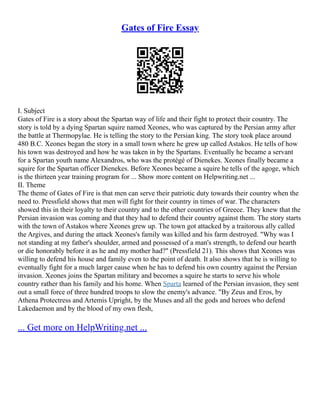The image features an online article with a white background. At the top, there's blue underlined and clickable text that reads "Gates of Fire Essay." Below this text is a black-and-white QR code. The article consists of two detailed paragraphs, marked with Roman numerals. The first paragraph, labeled "I. Subject," discusses the Spartan way of life and their fight to protect their country, outlining the essay’s main subject. The second paragraph, labeled "II. Theme," explains that the theme of "Gates of Fire" is about men fulfilling their patriotic duty towards their country in times of need. At the bottom of the article, there is another blue underlined hyperlink that says "Get More on HelpWriting.net." This structured layout includes prominent hyperlinks and a QR code, making it an informative and interactive piece on the Spartan-themed essay.